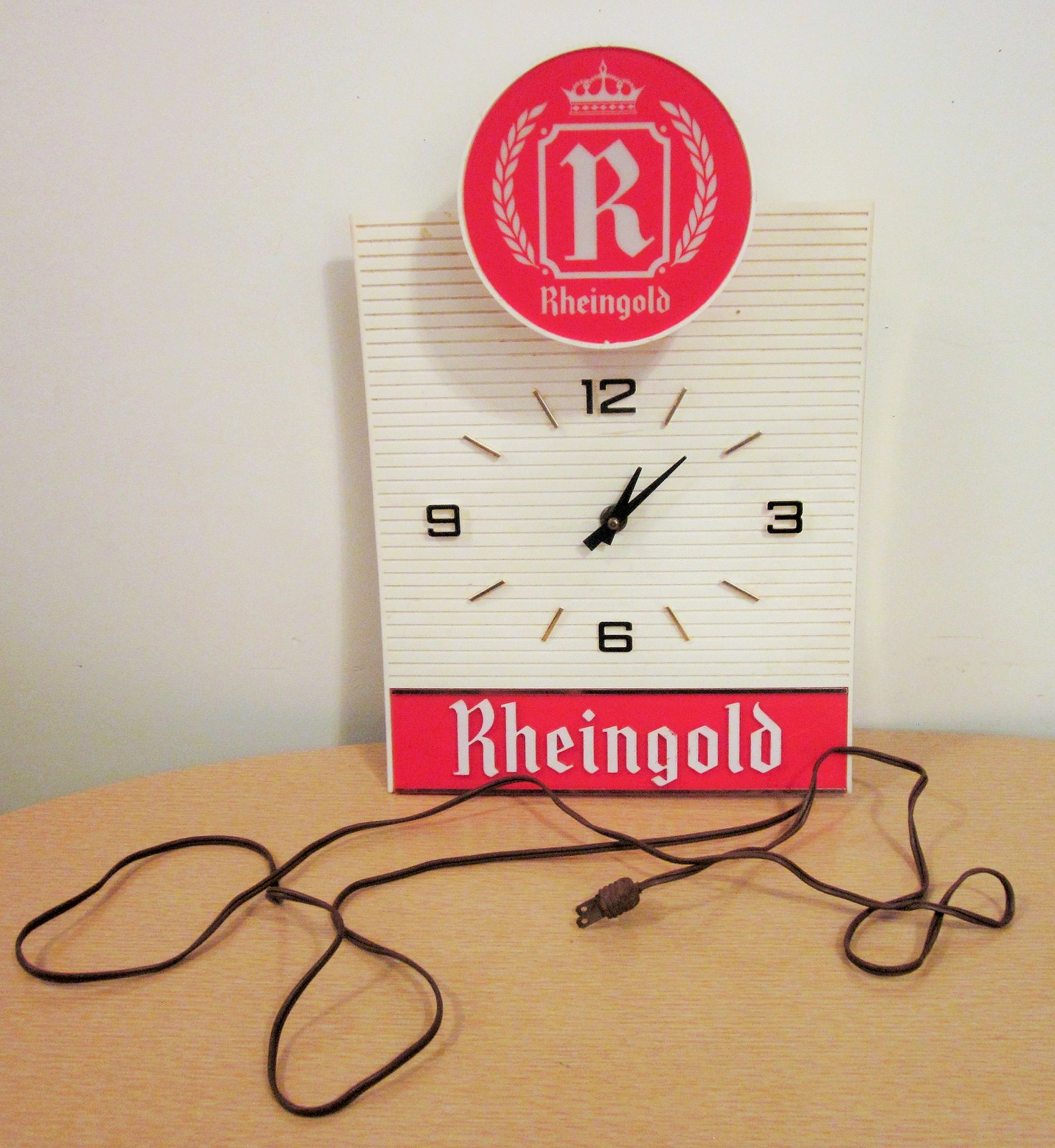This vintage-style photograph captures a carefully arranged scene with a sense of nostalgic charm. Dominating the bottom one-third of the image is a creamy solid table, providing a neutral foundation for the objects displayed. Propped up against a pristine white wall behind the table is a rectangular clock, which features a striking red border at its base with white text that reads "Rheingold." In front of the clock, an intricately curled long brown cord adds an element of visual interest. Atop the clock sits a round medallion adorned with a prominent, bold letter "R" set against a vibrant red background, with the word "Rheingold" inscribed in smaller print beneath it. The clock, displaying a time of 1:08, features two contrasting black arms indicating the hour and minute. This meticulously composed tableau offers a glimpse into a bygone era, rich with detail and texture.